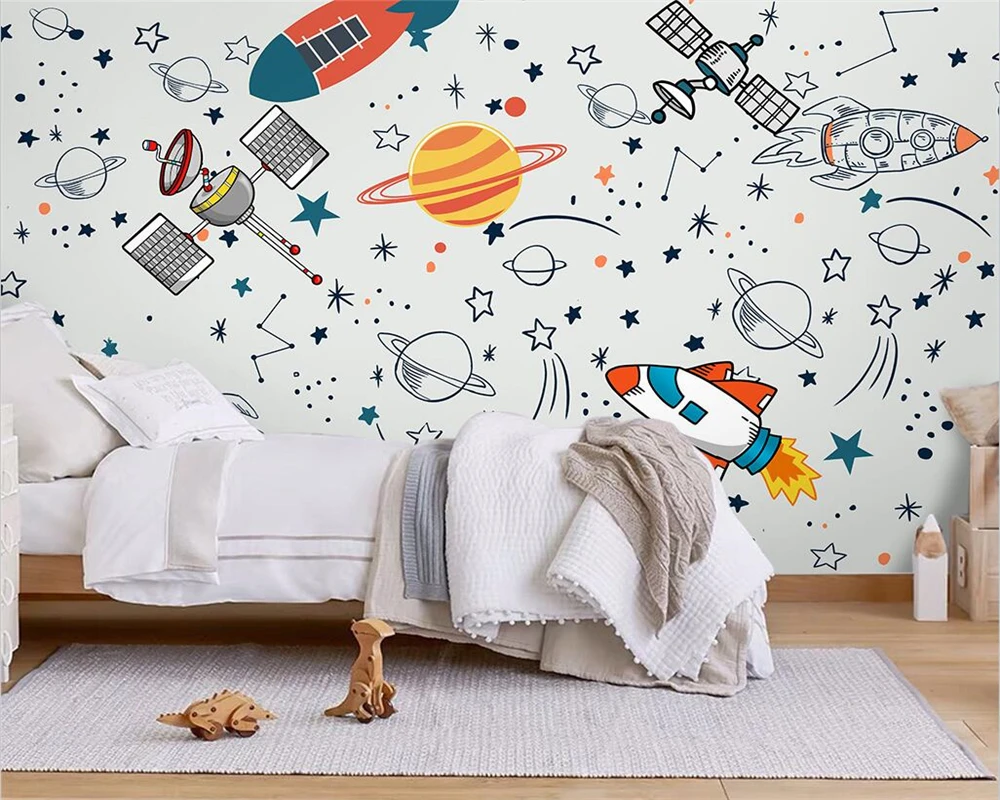The image depicts a young boy's minimalist bedroom with a prominent space theme. The walls are adorned with detailed illustrations of celestial objects, including planets with rings, various rockets, satellites, stars, constellations, and shooting stars. Most of the images are in black and white sketch style, but some feature bright colors—an orange and blue rocket, a white spaceship with orange tips, a red and blue rocket with fire, and a yellow and orange striped planet with rings. The room is neatly arranged, with a simple bed positioned on the left side against the wall. The bed has white bedding with multiple folded blankets in shades of beige, gray, and blue. The floor is a medium brown wood partially covered by a cream rectangular rug. On this rug, there are two wooden dinosaur toys with wheels, designed to be assembled and disassembled. On the right side of the image, there's a tall decorative white pencil and the edges of a couple of wooden boxes. The overall aesthetic is clean and organized, highlighting the vibrant space-themed illustrations on the wall.